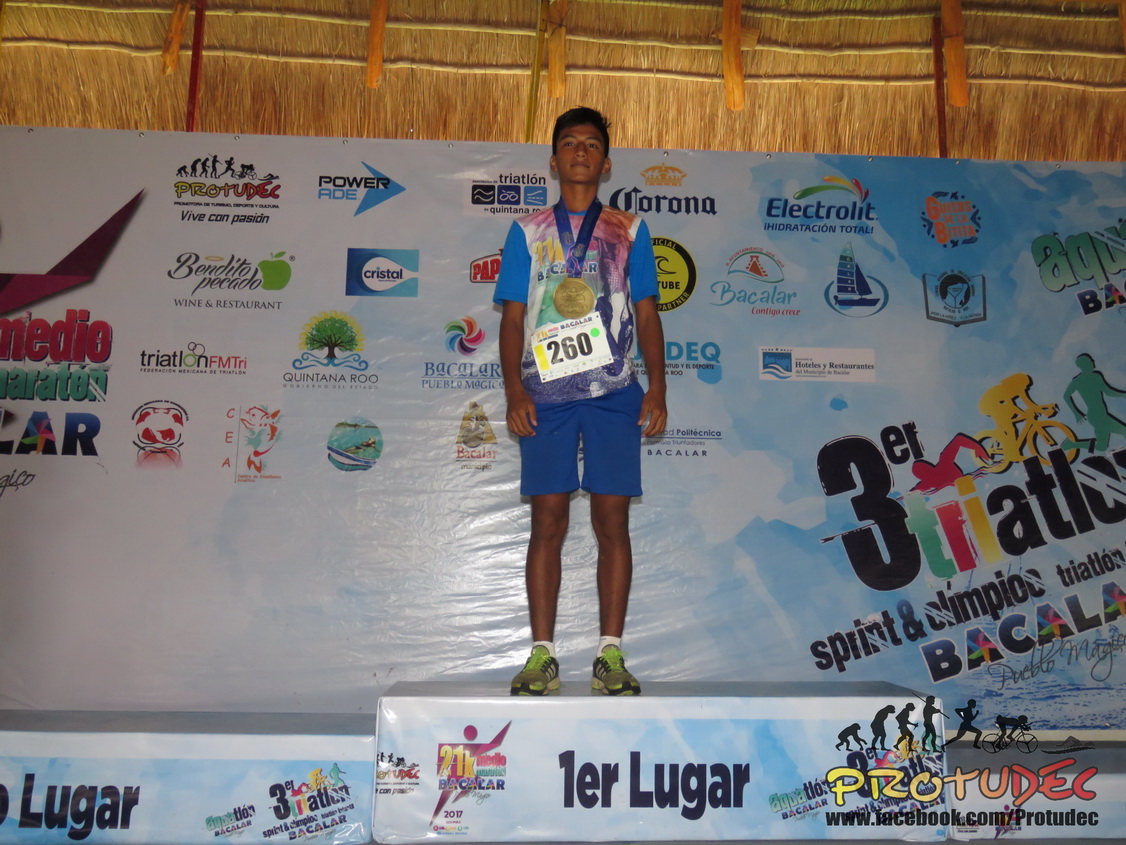The photograph captures a young man of possible Latino, Asian, or East Indian descent standing triumphantly on a stage or podium, illuminated in a setting with walls resembling straw, hay, or light wood. His short dark hair complements his blue shirt adorned with a myriad of colors, blue shorts, and bright green sneakers that appear slightly dirty. A large gold medal with a blue ribbon hangs proudly around his neck, signifying his victory in a race or competition. The runner’s bib on his shirt displays the number 260. The backdrop features a large, sky-colored banner with white clouds and ocean-themed designs, encompassed by numerous company logos, including Crystal, Papa John's, Corona, Bacalar, and Quintana Roo. An inscription on the banner indicates the event: the "3ER Triathlon, Sprint and Climb, Klimpiak Triathlon." Despite the visible indicators of his athletic accomplishment, he stands alone on the podium, with no other competitors in sight.